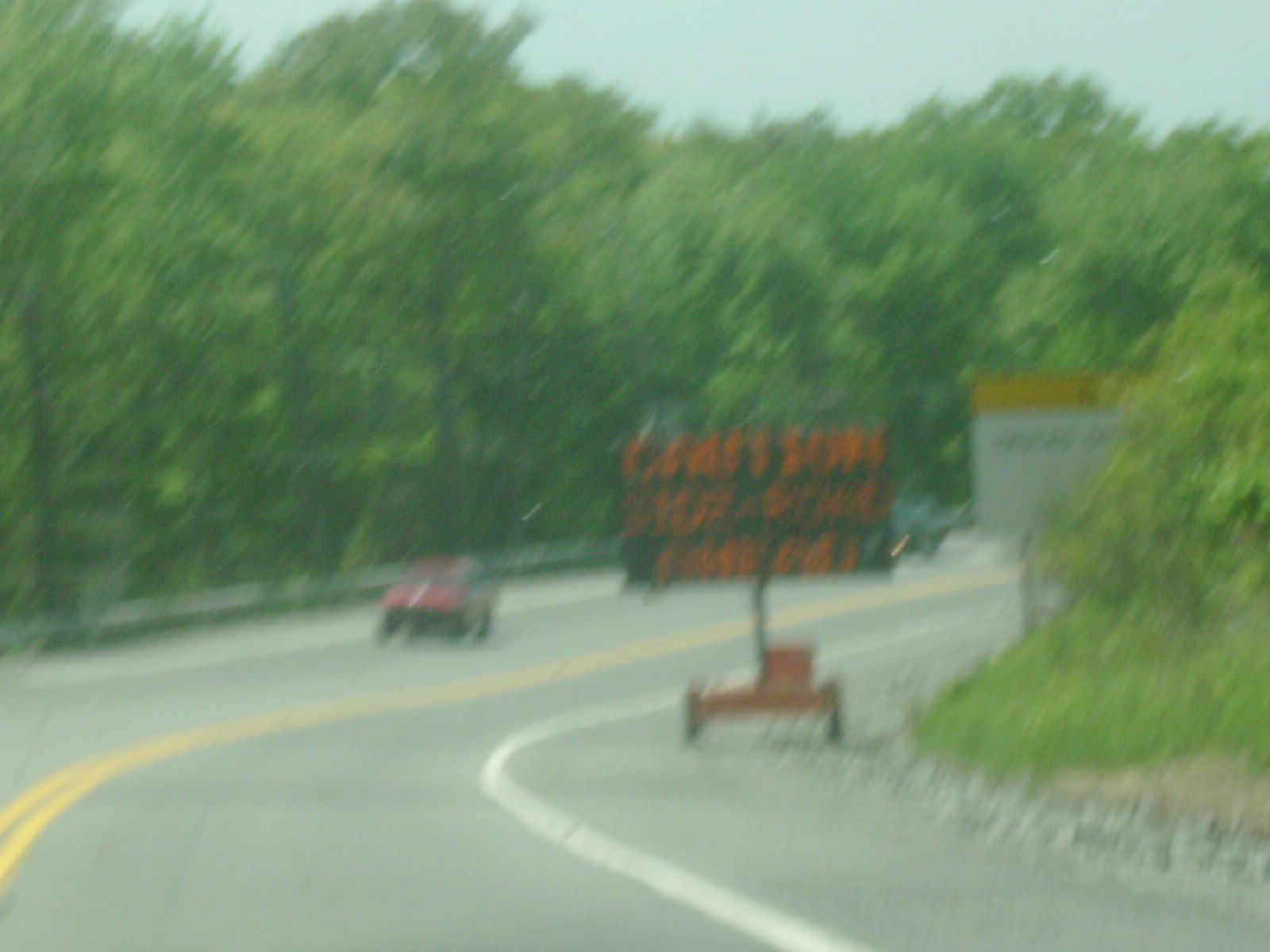The image is a very blurry photograph depicting a two-lane, paved road curving into the background, situated in a heavily wooded area lined with green trees. The road features white lines on either side and yellow lines in the center, enhancing the perception of its curve. In the foreground, a red vehicle, either a car or truck, is coming towards the viewer. On the opposite side of the road from the vehicle, there is a blurry construction sign with black backing and orange lettering at the base, suggesting caution; however, the specific wording remains illegible. Adjacent to this construction sign is another white sign with a yellow strip on top, but its text is equally unreadable due to the blur. A guardrail is visible in front of the trees, alongside both signs, ensuring safety between the road and the forested area beyond.